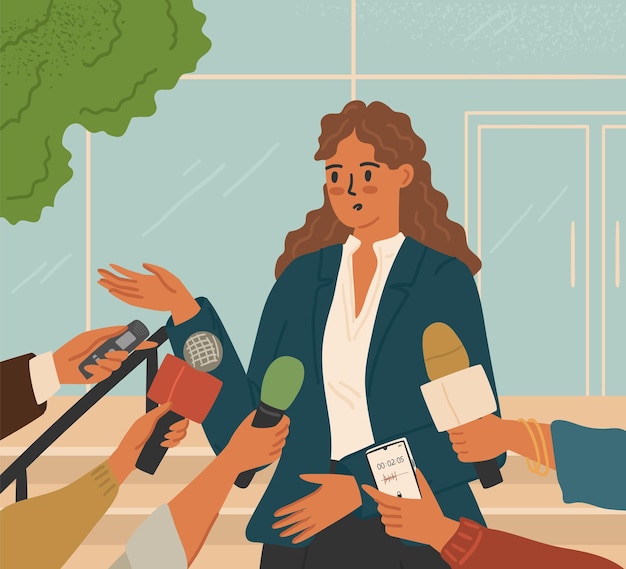This is a color illustration depicting a woman being interviewed by news reporters in a cartoon style. The woman is positioned in the center, with long, wavy brown hair cascading behind her shoulders and a solemn expression on her face. She has a tan complexion, black eyes, and subtle hints of blush on her cheeks. She is dressed in a white V-neck shirt under a navy blue blazer and appears to be wearing a gray skirt or pants, although the bottom half of the image is not fully visible. Her left hand is raised, while her right hand rests at waist level.

In the foreground, numerous arms are extended towards her, holding various recording devices including microphones, tape recorders, and a cell phone displaying a timer reading 00:02:05. 

The background features a white-blue building with glass windows and doors, highlighted by white block stripes creating a structured design. In the upper left corner, a green tree with dark green squiggles and dots adds a touch of nature to the scene. The illustration employs bold, sleek lines for a clean and simple, yet stylized aesthetic.